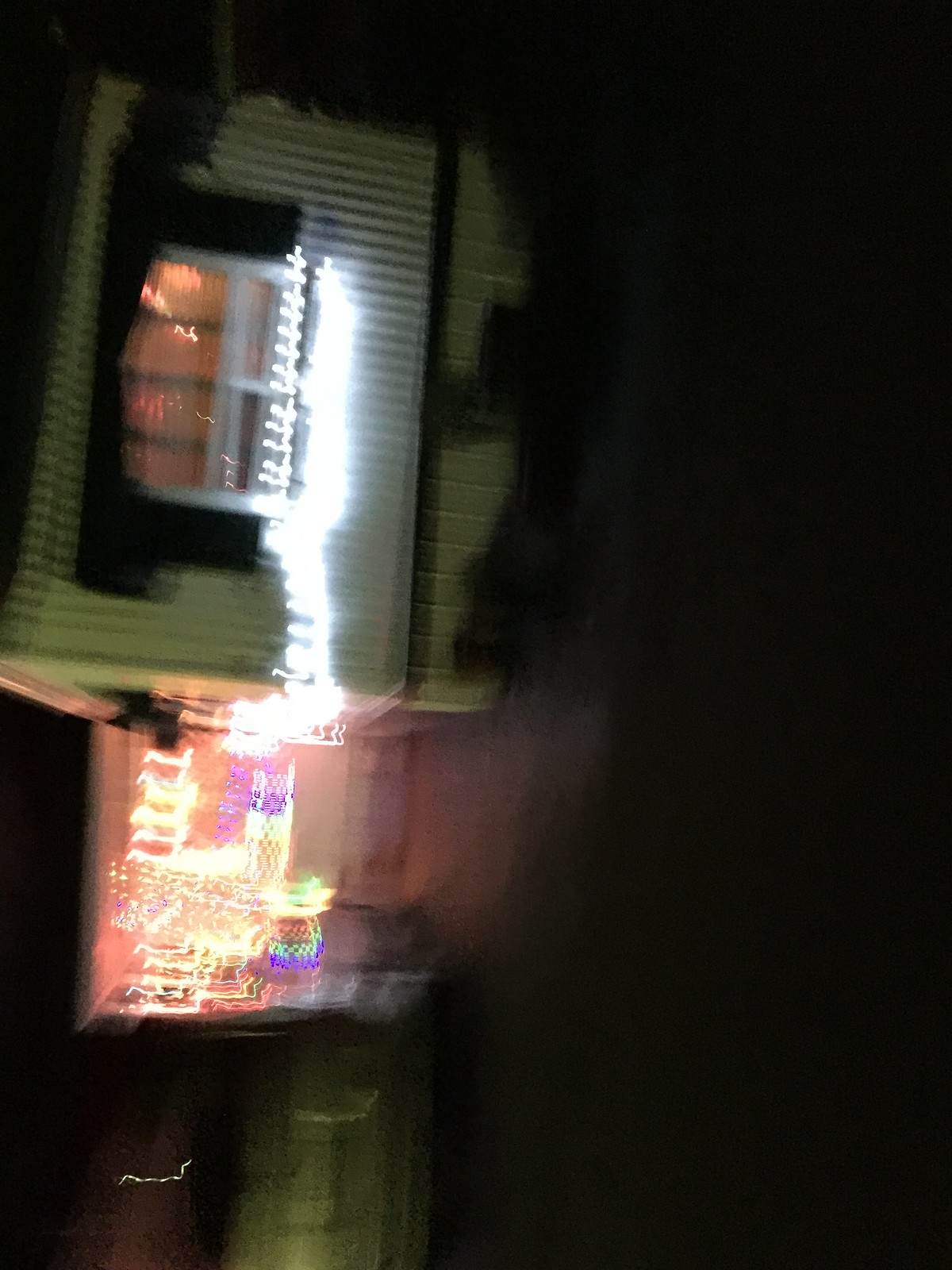A blurry nighttime photograph of a house turned sideways, requiring you to tilt your head to the left to view it properly. The house, painted a yellowish hue with dark shutters framing the windows, features a warmly lit cove at the front door. The right side of the image shows a bedroom window, while further left, the house extends outward slightly. Decorative lights around the front entrance create a scatter of light trails, adding to the photo's disoriented feel.